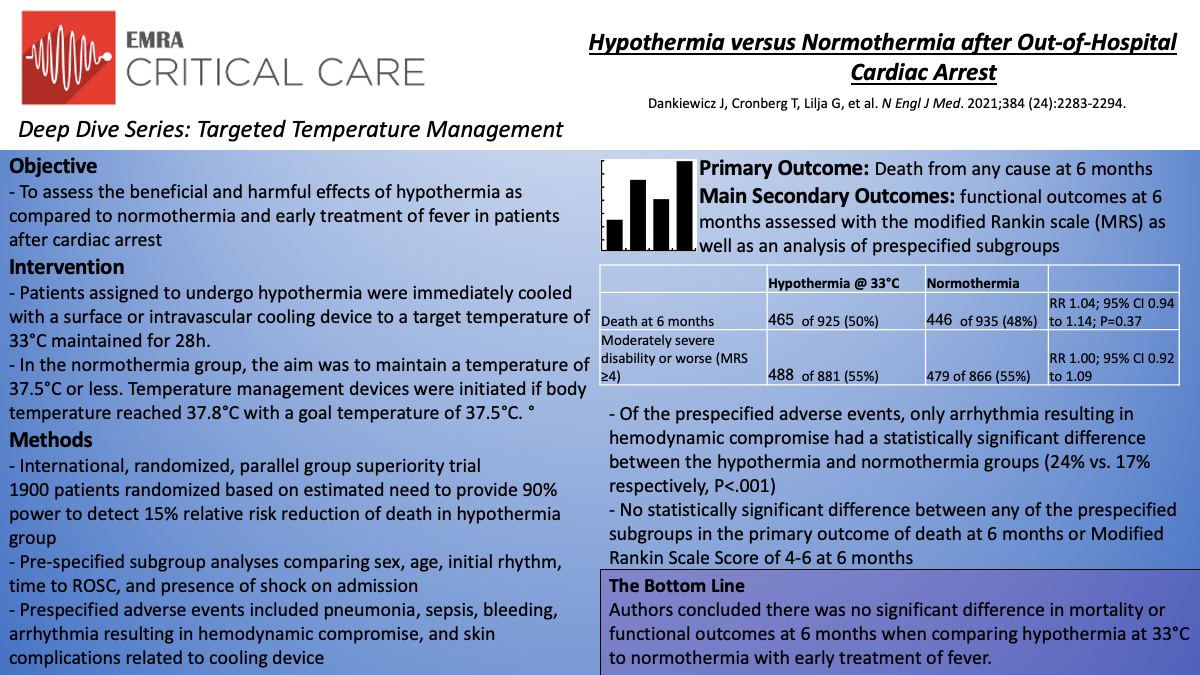This instructive PDF slide, likely designed for an educational brochure or poster, presents a detailed overview of Targeted Temperature Management in critical care. The slide is labeled "EMRA Critical Care Deep Dive Series" and prominently features the topic "Hypothermia versus Normothermia After Out-of-Hospital Cardiac Arrest." 

The left side of the slide includes a red square with lines resembling a heartbeat monitor, and beneath it, core headings such as Objective, Intervention, and Methods are outlined in black text on a blue background. The objective is to assess the beneficial and harmful effects of hypothermia compared to normothermia and early treatment of fever in post-cardiac arrest patients. The intervention details specify that patients undergoing hypothermia were cooled to 33 degrees Celsius using a surface or intravascular device for 28 hours, while the normothermia group's target temperature was maintained at 37.5 degrees Celsius, with cooling initiated if the body temperature reached 37.8 degrees Celsius.

On the right side, the heading "Hypothermia versus Normothermia After Out-of-Hospital Cardiac Arrest" is presented along with a citation: Dankwitz J., Kramberg T., Lilja G., et al., published in the New England Journal of Medicine, 2021, 384(24): 2283-2294. This section includes a bar chart showing different outcomes— the first bar being the shortest, the second doubling in size, the third shorter than the second, and the final bar being the tallest. Headings like Primary Outcome, Main Secondary Outcomes, and The Bottom Line summarize the findings, showing no significant difference in mortality or six-month functional outcomes between hypothermia at 33 degrees and normothermia with early fever treatment. 

The blue box on the right also includes a table comparing outcomes related to hypothermia at 33 degrees Celsius and normothermia, specifically measuring death at 6 months and moderately severe disability or worse, defined as MRS ≥ 4. The Bottom Line is highlighted in purple, reinforcing the study's conclusion.

Overall, the slide combines detailed textual information with visual aids to effectively communicate critical findings and methodologies related to Targeted Temperature Management in a post-cardiac arrest scenario.